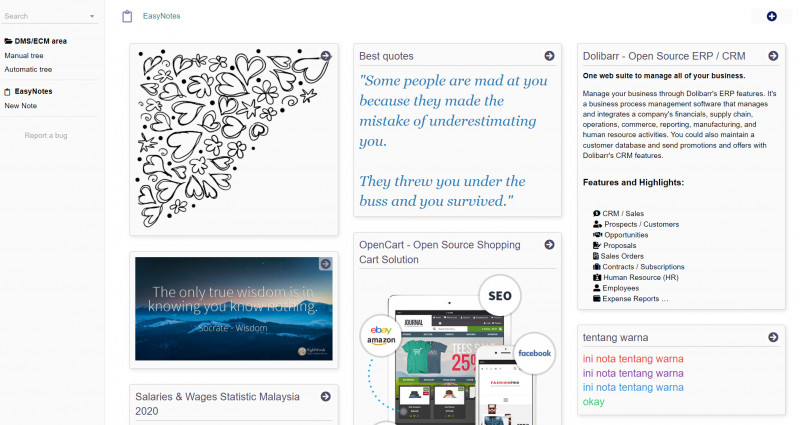This image is a collage consisting of six differently sized squares and rectangles, each featuring distinct content against an off-white background. Moving systematically from the top left to the bottom right:

1. The top left section showcases a white rectangle filled with hand-drawn black hearts. These hearts are scattered across the area, especially concentrated along a diagonal line running from the top left corner to the bottom right corner. Interspersed among the hearts are small sketches of flowers and dots, adding to the whimsical aesthetic.

2. Positioned next to it, in the top middle, is a small square with the title "Best Quotes." Below the title, in blue text, is an inspirational quote reading: "Some people are mad at you because they made the mistake of underestimating you. They threw you under the bus, and you survived."

3. The top right section displays an advertisement for a business solutions product titled "Dolibarr Open Source ERP & CRM." This advert lists various features of the product, highlighting its utility for business management.

4. In the bottom left, there is a poster featuring another inspirational quote, although the exact text of the quote is not specified in the description.

5. The center of the bottom row contains an advertisement for an open-source shopping cart solution known as "OpenCart." It appears to be a promotional poster detailing the benefits or features of this e-commerce platform.

6. Finally, in the bottom right corner, there is a small square titled "Tentang Warna." The phrase "Tentang Warna" is repeated three times in different colors, adding a visually attractive element to the collage.

The cohesive off-white background ties the pieces together, creating a visually diverse yet unified presentation.